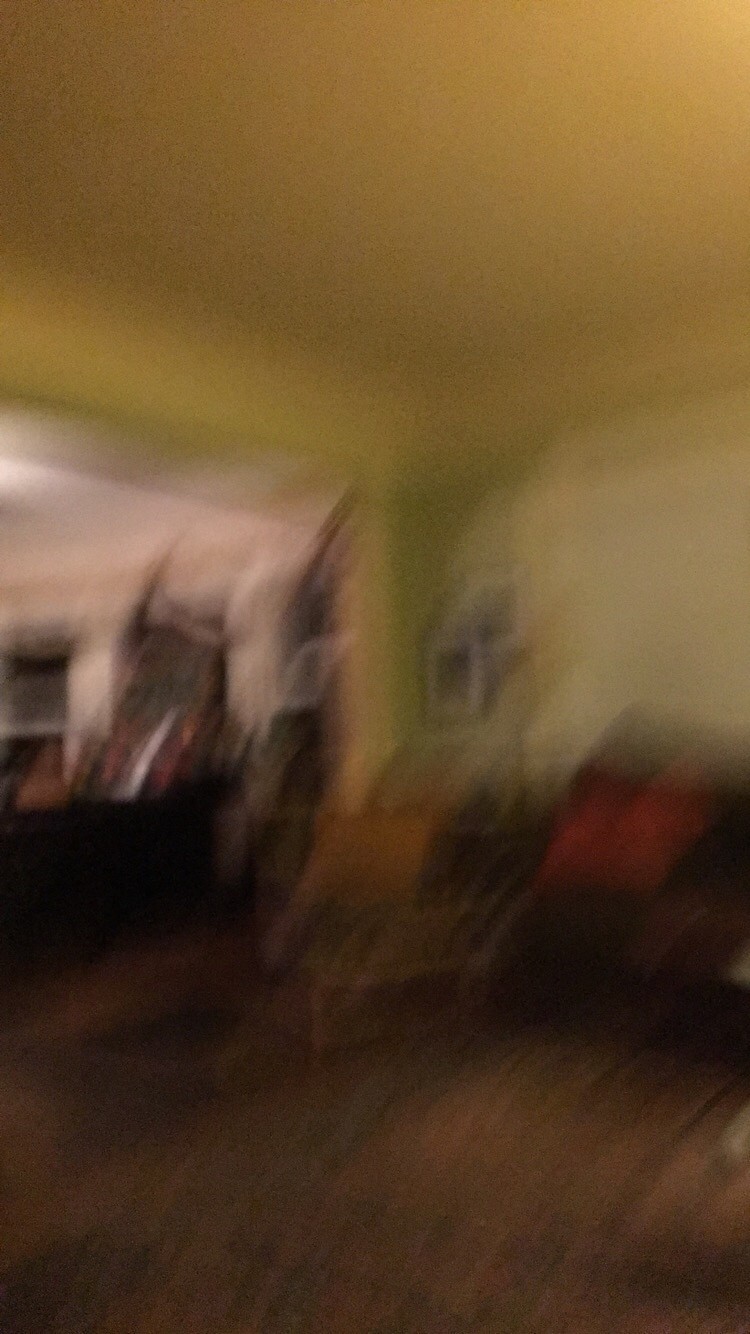This extremely blurry image, likely taken by someone moving within a home, captures an indoor scene with various pieces of furniture, though details are hard to discern. At the core of the picture appears to be a living room that transitions into a larger space, possibly a dining room or great room, characterized by an open concept with a separating wall. Dominating hues are a greenish tint for the walls and a tan or off-white ceiling, tinged with grey and brown tones.

In the foreground, a brown couch with a prominent red pillow and a brown chair featuring a yellow pillow can be detected. Central to the living area is a brown carpet. To the right, amidst the fuzziness, you can spot a large red cushion and a table. Observers have noted pictures hanging on the greenish walls. The living room precedes a larger area through a broad doorway or archway, and beyond this, multiple windows are visible, suggesting an open, well-lit space, possibly overlooking a bar area. The overall image gives a sense of moving through a cozy, albeit indistinct, home environment.